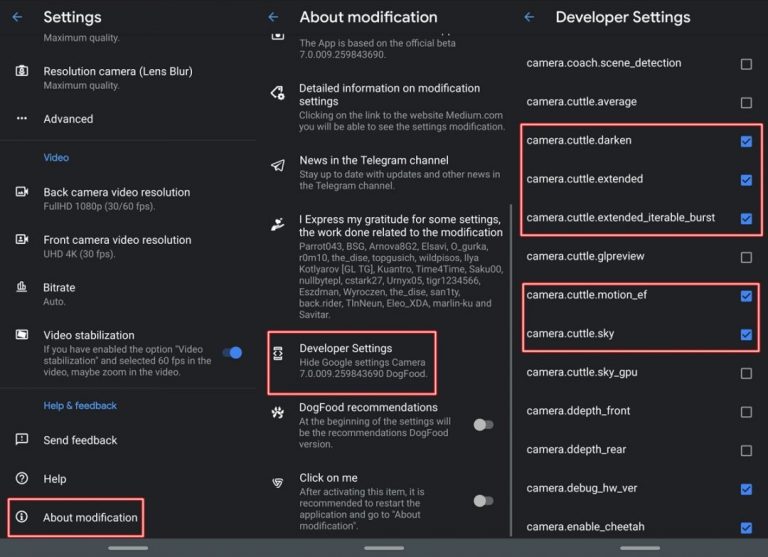The screenshot captures the settings interface of a tablet or smartphone application, characterized by its black background adorned with white and gray textual elements. The interface is divided into three distinct columns. 

**Left Column:**

- **General Settings:**
  - **Title:** Settings (in white)
  - **Subtitle:** Maximum Quality (in gray)
  - **Options:**
    - **Resolution (Lens Flare):** Maximum Quality
    - **Advanced Settings:** Represented by three ellipses
    - **Video Settings (in blue):**
      - **Back Camera Video Resolution:** Full HD, 1080p (30/60 FPS) (in gray)
      - **Front Camera Video Resolution:** UDH, 4K (30 FPS)
    - **Additional Options:** Bitrate, Video Stabilization, Send Feedback, Help, About Notification (highlighted with a red rectangle and an eye icon)

**Middle Column:**

- **About Notification:**
  - **Application Information:** Based on the official beta 7.0.009.259.84.43690
  - **Details:**
    - Detailed information on notification settings
    - News and Telegram Channels
    - Acknowledgment section for work related to notifications

- **Developer Settings:**
  - **Options:** Dog food recommendations, clickable option labeled "Click on me"

**Right Column:**

- **Developer Settings (highlighted with a blue arrow):**
  - **Unchecked Options:**
    - camera.coach.scene_detection
    - camera.cuddle.average

  - **Highlighted with Red Rectangles and Selected:**
    - camera.cuddle.darken
    - camera.cuddle.extended
    - camera.cuddle.extended.irritable_burst

  - **Outside Red Rectangle and Unchecked:**
    - camera.cuddle.GL_preview

  - **Inside a Red Rectangle and Selected:**
    - camera.cuddle.motion_EF
    - camera.cuddle.sky

  - **Outside Red Rectangle and Unchecked:**
    - camera.cuddle.sky_GPU
    - camera.DD.depth_front
    - camera.DD.depth_rear

  - **Selected Options:**
    - camera.debug.HW_VAR
    - camera.enable.cheetah_T-H-E-E-T-H-H

This organized layout and comprehensive detailing of settings enable easy navigation and customization of the application’s features.